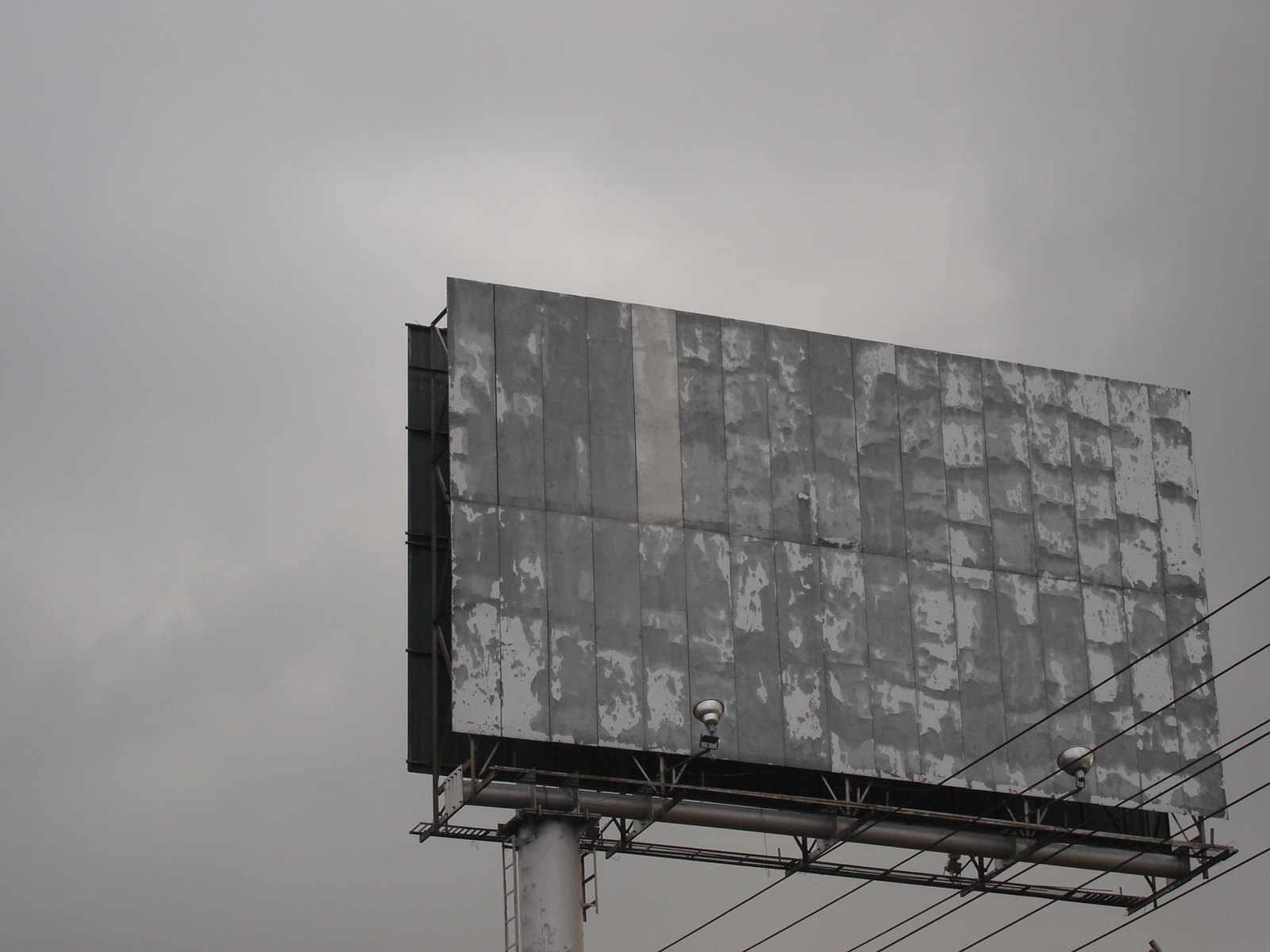This black-and-white photo captures a large, weathered, two-sided billboard standing against a backdrop of a mixed white and gray overcast sky. The photograph is taken from a slight angle, looking up at the billboard, with the imposing steel beam and attached ladder visible to the left of center. The steel beam, extending up from the bottom of the image, supports the vacant billboard, which is marked with varying shades of light and dark gray patches where advertisements once clung. Below the billboard, about an inch in from both the left and right edges, are two white spotlights aimed upwards, though unlit. Diagonally crossing the bottom right-hand corner of the image are four black power lines, adding to the stark, somber tone of the scene.